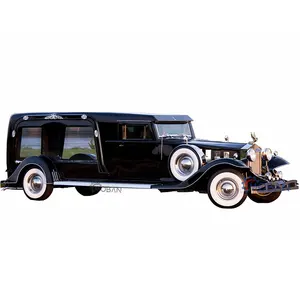The image showcases an old-styled, luxury vehicle from the early 1900s, likely a model reminiscent of a Rolls-Royce. The car, painted entirely in a glossy black with white trimming, features a boxy, elongated shape. Notable elements include a gold front grille and elegant lights, with an eagle emblem in gold positioned at the front where a brand symbol is typically found. The vehicle has four white side tires, with a spare tire mounted between the front fender and the side of the car, beside the main passenger area. The car's rear end, which looks similar to a hearse, has two large windows that intriguingly appear to depict a nature scene of grass and water. The interior is partially visible, showing brown trimmed seats. The entire scene is set against a completely white backdrop.